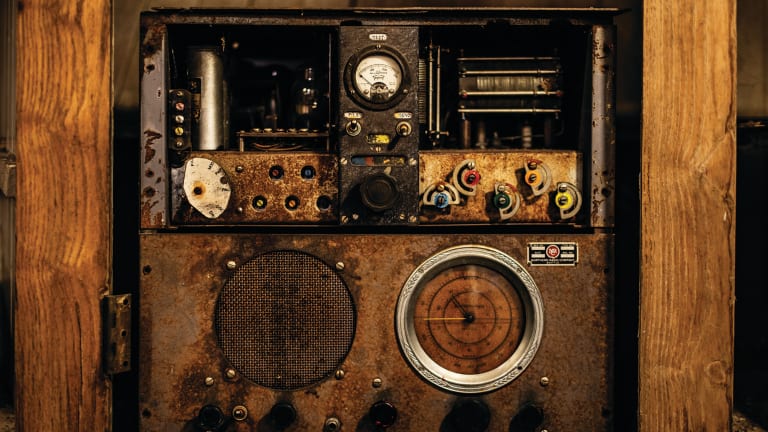This photograph captures a close-up view of an antique radio, featuring a rustic and distressed metal surface framed by wood. Dominating the upper section is a small, circular gauge with a needle currently pointing to zero, resembling a compass. Below this, on the right, is a larger, clock-like tuner gauge, flanked by a cluster of colorful adjustment knobs in blue, red, green, orange, and light yellow. Adjacent to the tuner gauge, there is a smaller speaker covered with cloth. The radio, possibly an old RCA model, shows considerable wear, with visible rust adding to its vintage charm. The upper left section reveals what appears to be radio tubes, further emphasizing the device's bygone era and mechanical complexity.